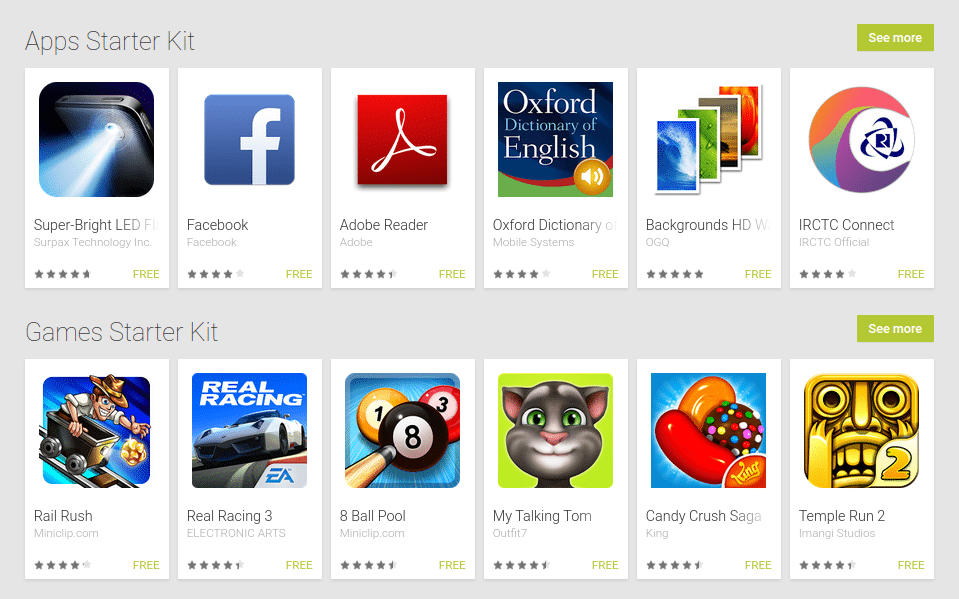This image is a screenshot of an app store interface showcasing an "Apps Starter Kit" and a "Games Starter Kit". The layout is marked by a light gray box framing the entire image. In the top right corner, there's a lime green button with white text that says "See More." 

Below this section, a list of different free apps is displayed, each app residing within its white square. The apps in this initial list include:

1. Super Bright LED Flashlight (rated between 4 and 5 stars)
2. Facebook (rated between 4 and 5 stars)
3. Adobe Reader (rated between 4 and 5 stars)
4. Oxford Dictionary (rated between 4 and 5 stars)
5. Backgrounds HD (rated between 4 and 5 stars)
6. IRCTC Connect (rated between 4 and 5 stars)

Following this, the "Games Starter Kit" section is presented, also accompanied by a lime green "See More" button on the far right. This section outlines a list of six free games, including:

1. Real Racing 3
2. 8 Ball Pool
3. My Talking Tom
4. Candy Crush Saga
5. Temple Run 2

Each app and game is visually represented by its logo or associated image, reinforcing the distinction between productivity/social media applications and gaming applications.